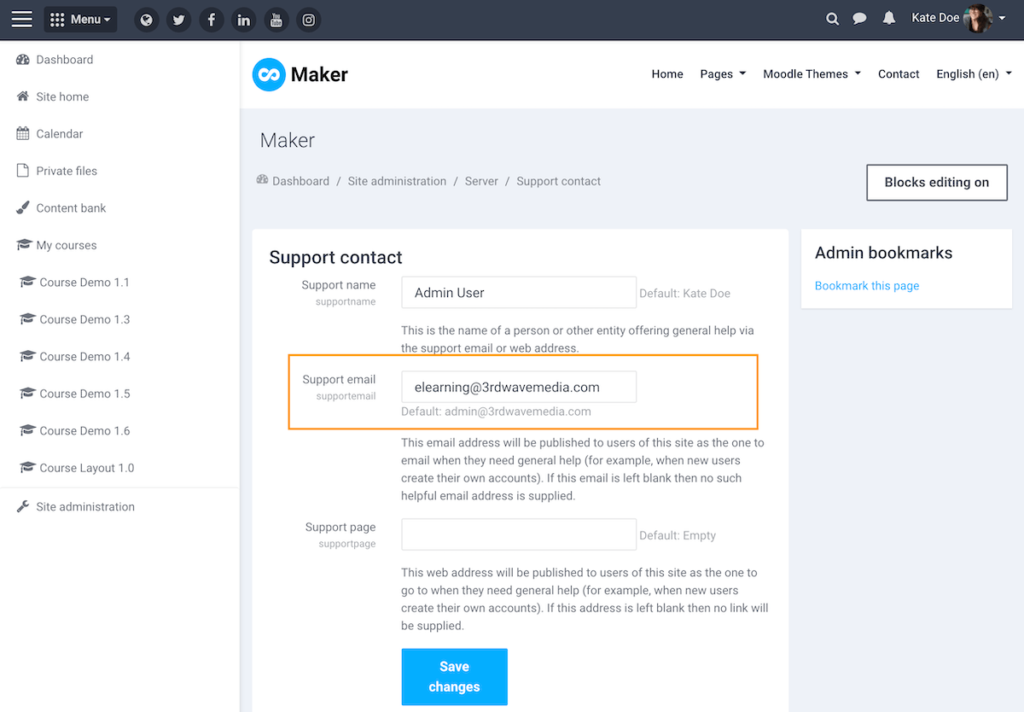A detailed, descriptive caption for the given image could be:

"This screenshot displays an e-learning dashboard interface. Dominating the left side of the screen is a vertical side panel listing various topics in a sequential order, starting with 'Dashboard' at the top and progressing through 'Site Home,' 'Calendar,' 'Private Files,' 'Content Bank,' followed by multiple demo courses denoted as 'Course Demo 1.1' through 'Course Demo 1.6' and 'Course Demo 1.0.' Towards the bottom of this panel, there is an option titled 'Site Administration,' marked with a small wrench icon.

Central to the display, the topmost section highlights the word 'Maker,' accompanied by a white infinity symbol within a blue circle. Below this header, in lighter gray text, are navigational breadcrumbs reading 'Dashboard / Site Administration / Server / Support Contact.' This section reveals support-related information, including 'Support Name: Admin User' and 'Support Email: elearning@thirdwavemedia.com,' with the email address enclosed within an orange-bordered box. Additionally, beneath this, a notification clarifies that this email address will be publicly accessible on the site for users seeking general help. This screenshot effectively illustrates a help support contact page within an educational platform."